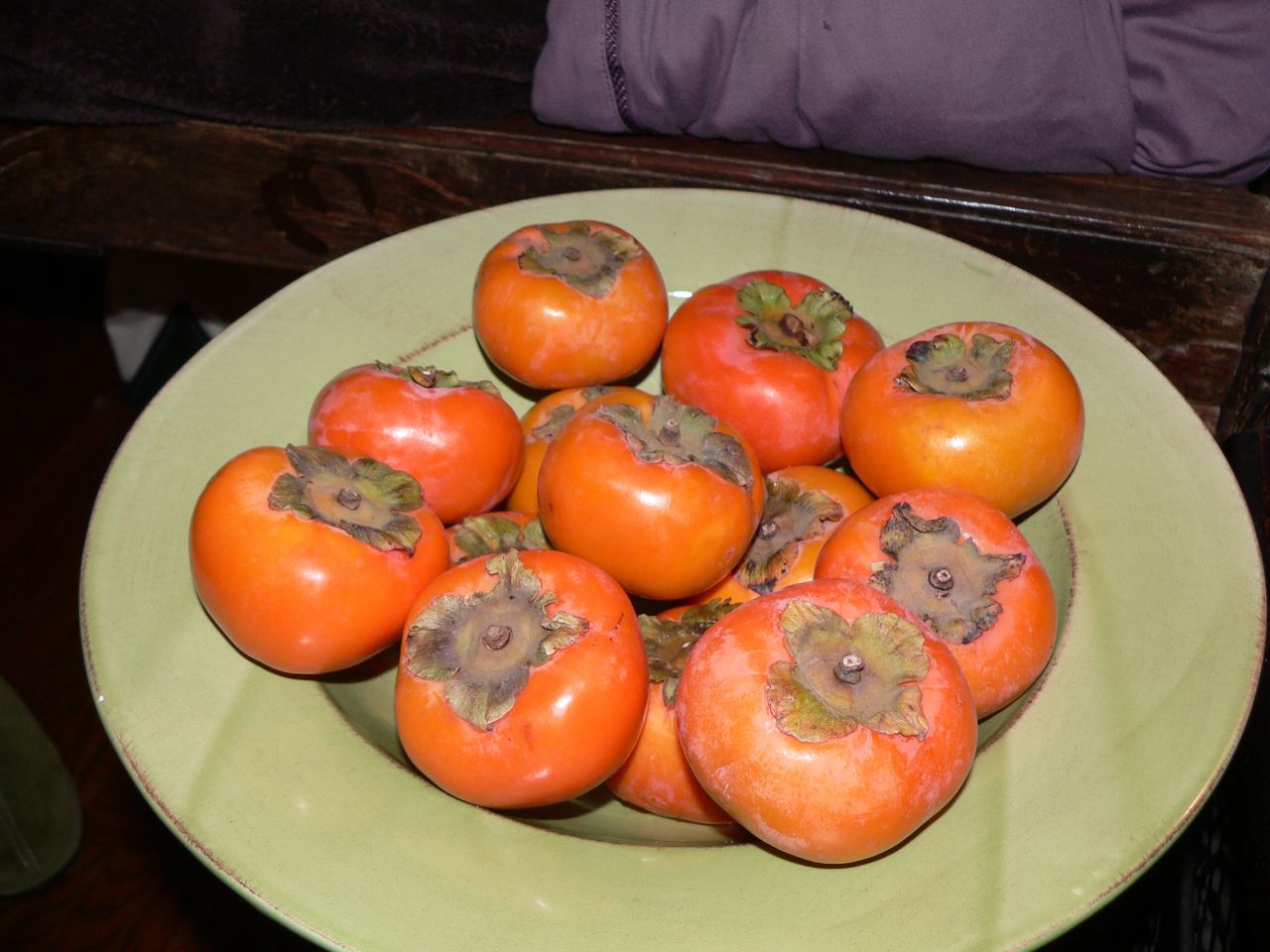The image shows a shallow, sage-green bowl with a wide brim containing approximately a dozen tomatoes. These tomatoes are an orangish-red hue, transitioning to a reddish-orange color, indicating ripeness, with some brownish tones. The tomatoes still have the leafy stems attached, which are dried up and crumpled, with a greenish-grayish to purplish tinge. The bowl rests on a dark wooden surface, possibly a table, and in the foreground, a slightly balled-up purple sheet is partially visible. The lighting in the image is somewhat dim, casting soft reflections on the smooth, shiny surfaces of the tomatoes. The combination of elements in the foreground and background suggests a cozy, rustic scene.